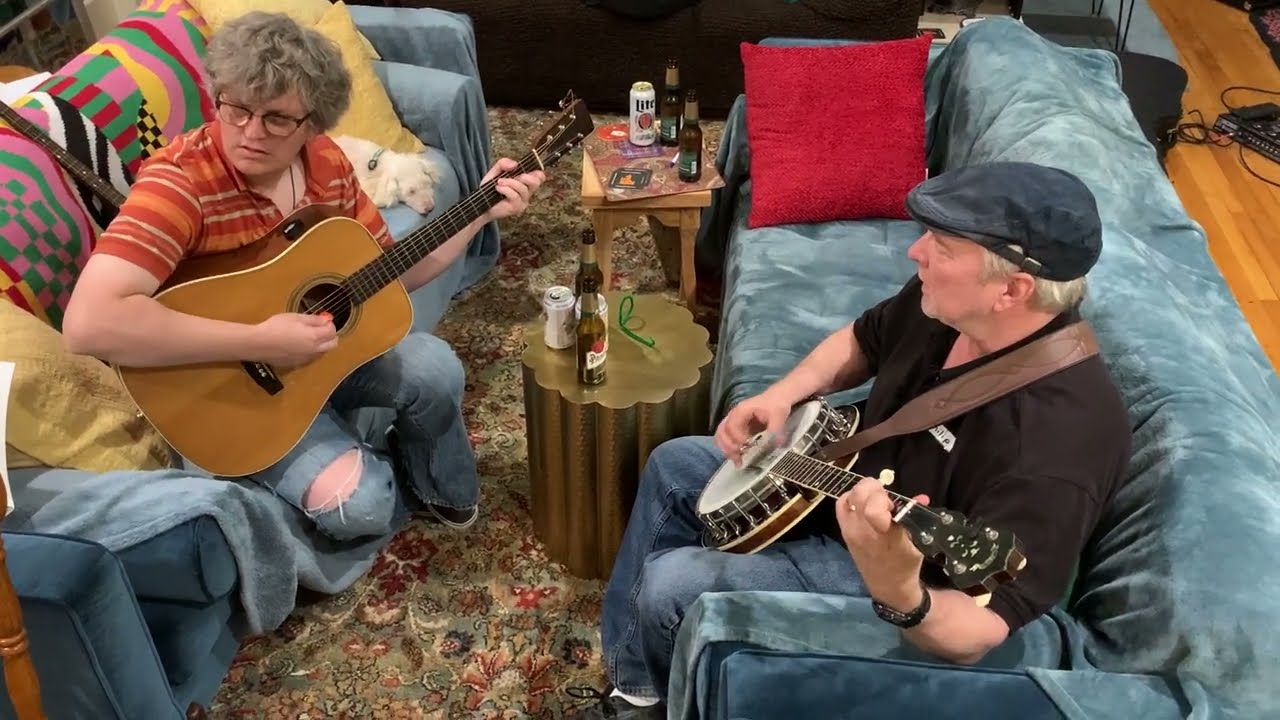In an inviting living room setting adorned with vibrant textiles, two individuals—both musicians—are seated on facing sofas, each covered with blankets. The sofa on the left features a row of pillows along the back and is occupied by a woman wearing an orange polo t-shirt and green-blue jeans, strumming a traditional guitar. Opposite her, an older man in a black t-shirt and blue jeans plays a banjo on a couch with a single pillow at one end. Between them, a coffee table and a stand are laden with various alcoholic beverages. The room is accented by a textured carpet with psychedelic, flowery patterns in reds, pinks, and purples, further enriching the cozy, indoor ambiance as the duo shares a musical moment.